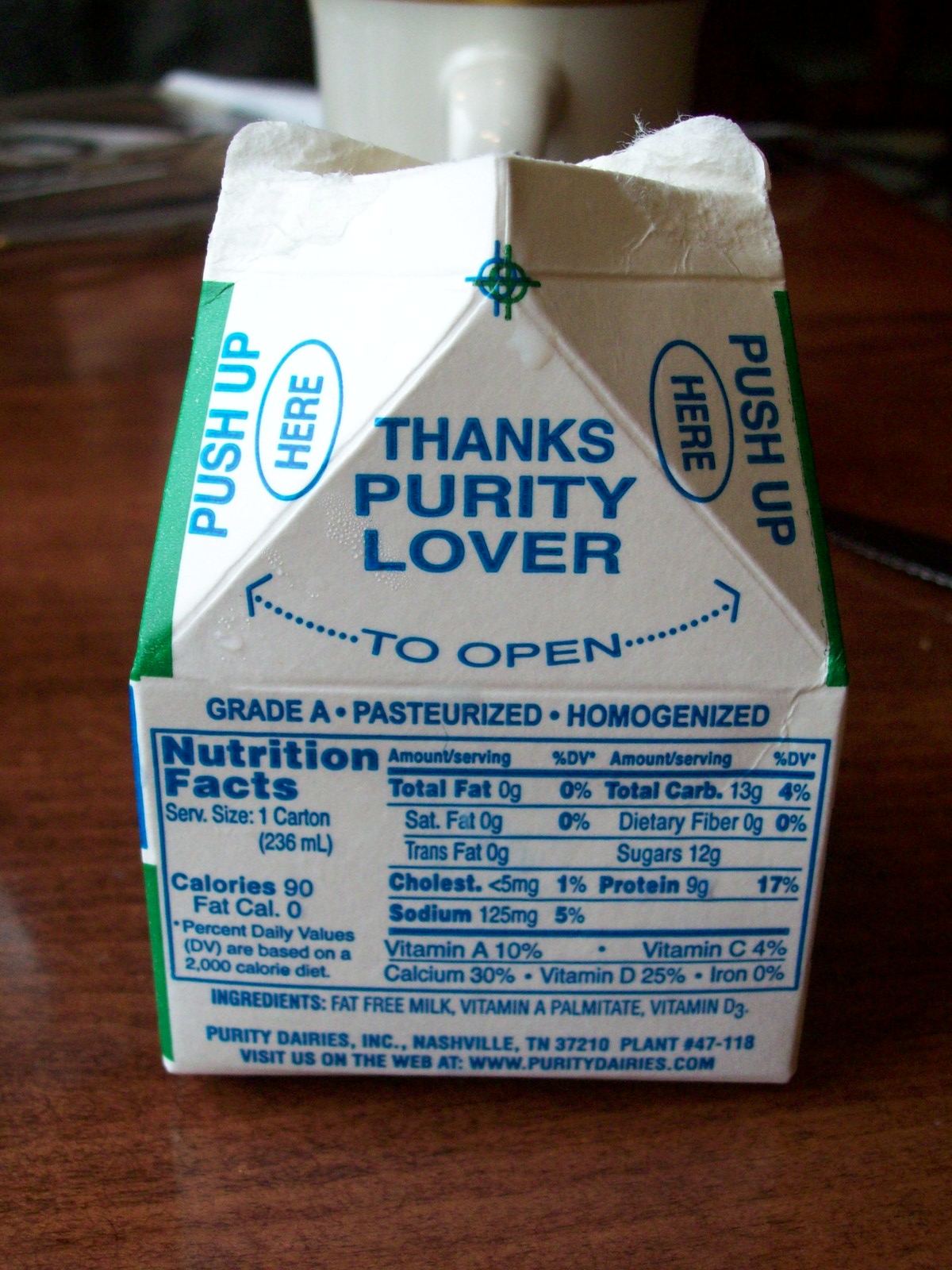This close-up photograph captures a small, mostly white cardboard milk carton accented with dark green edges and blue lettering, prominently featuring phrases like "PUSH UP HERE" and "THANKS, PURITY LOVER." The carton stands on a polished, dark brown wooden desk, streaked with darker shades, adding texture and richness to the surface. To the right center of the image, a white ceramic mug with a handle, partially obscured by the milk carton, adds to the composition. Blurry objects, likely papers, are visible in the left-hand corner.

The milk carton is opened at the top, revealing a triangular spout designed for pouring. Detailed nutritional information is visible on the back, including values for calories, fat, cholesterol, sodium, vitamins, and ingredients listed as fat-free milk, Vitamin A Palmitate, and Vitamin D3. The label also reveals that the product is Grade A, pasteurized, homogenized milk produced by Purity Dairies, Inc., located in Nashville, Tennessee, with a plant number 47-118. The website www.PurityDairies.com is also indicated.